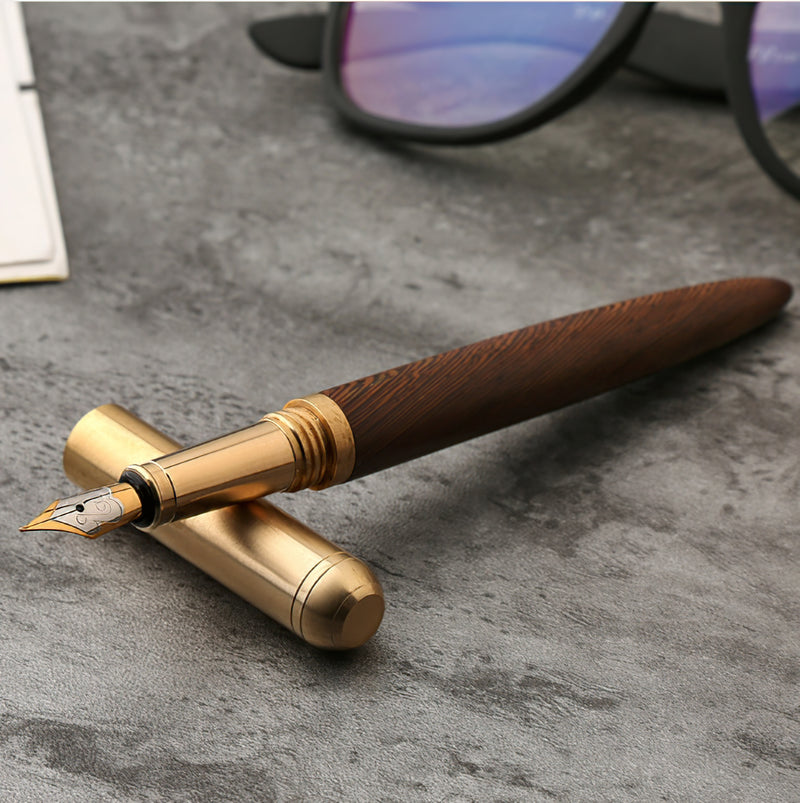This color photograph in a square format focuses on a fountain pen positioned on a dark gray granite or concrete-like table with a subtle marbled design. The pen, slightly angled with the top portion pointing towards the upper right and the ink point towards the lower left, features a dark wood grain barrel with intricate brown and black patterns. The capped portion is brass-colored, and the pen's metallic tip displays both gold and silver filigree. The fountain pen rests on its brass cap, which is aligned in the opposite diagonal direction. In the upper right corner of the image, partially cropped, are a pair of black sunglasses with blue reflective lenses. In the upper left corner, another partially cropped element is visible—presumably a white book or document. The photograph's style emphasizes photographic realism and detailed product representation.